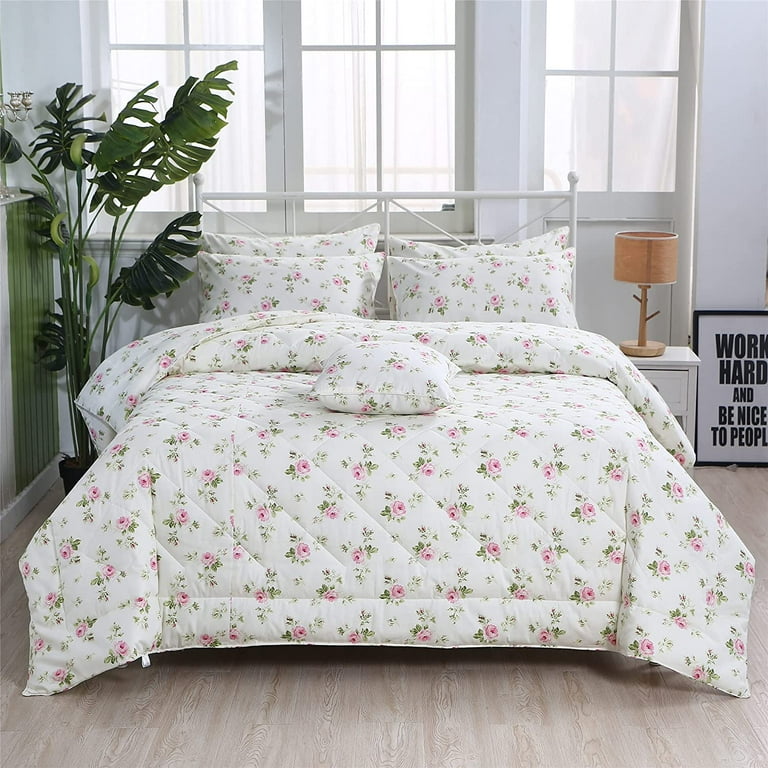The image depicts a serene white-walled bedroom featuring light gray laminate wood flooring. In the middle of the room stands a full-sized, neatly made bed with a white metal frame. The bed is dressed in a white comforter adorned with pink flowers and green leaves, which elegantly drapes down both sides. Four rectangular pillows, in matching white and pink floral cases, are stacked neatly at the head of the bed. Centered among them is a small square pillow with a white case decorated with pink flowers.

To the left of the bed, a potted artificial plant with large green palm leaves adds a touch of greenery to the room. The right side of the bed comprises a white side table with a small brown-shaded lamp on top. On the floor next to the side table rests a framed sign that reads, "Work hard and be nice to people."

The room is well-lit, thanks to several windows with white frames located in the background, hinting at an adjoining space adorned with sheer white curtains. The thoughtful arrangement and consistent color scheme contribute to the room's tranquil and welcoming atmosphere.